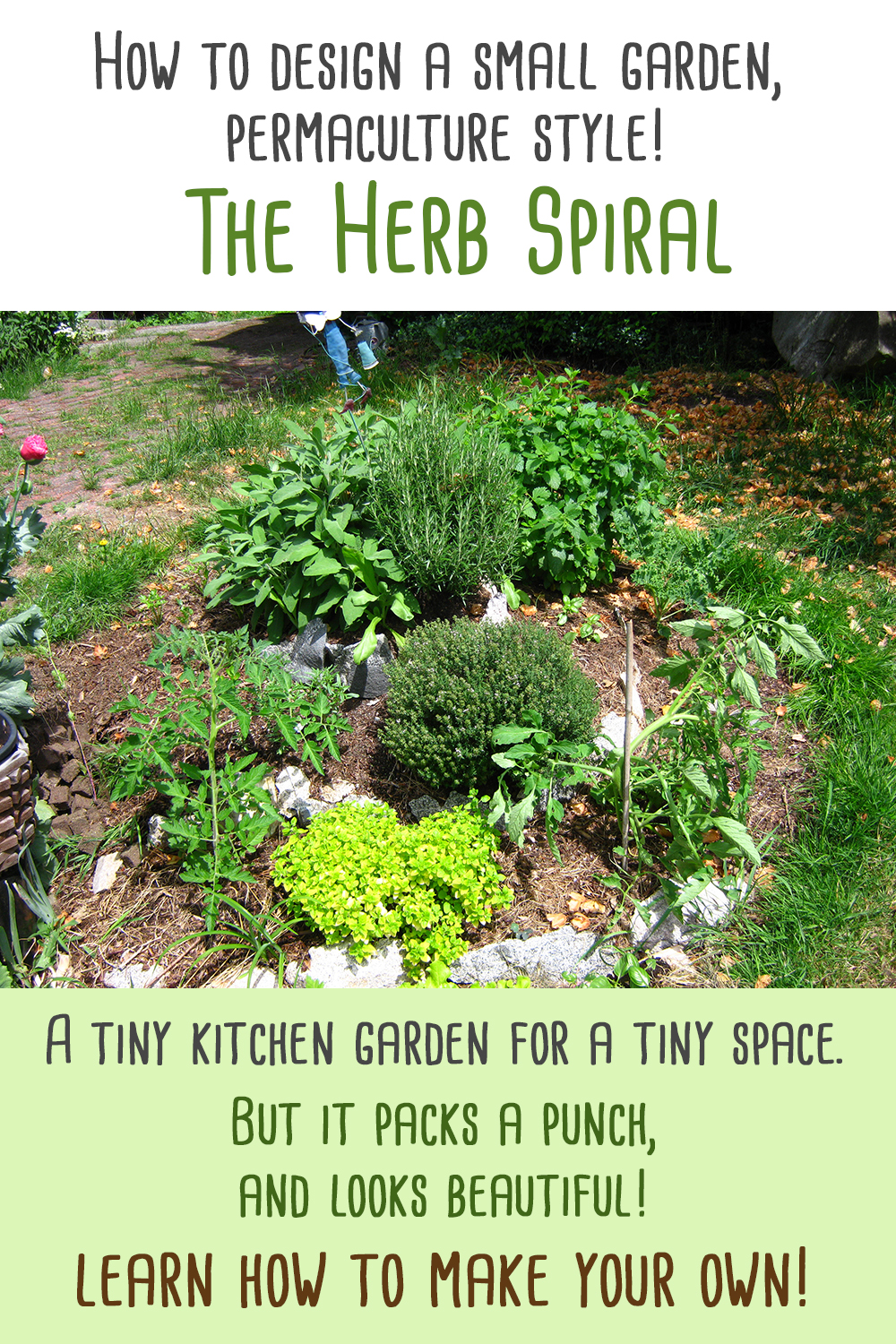The image appears to be an introductory page from a pamphlet or book about garden design, specifically focusing on creating a small, permaculture-style herb garden called "The Herb Spiral." At the top, it reads "How to Design a Small Garden, Permaculture Style," in a font that mimics a handwritten style, followed by the title "The Herb Spiral" in larger green lettering. The central photograph showcases a beautiful herb garden arranged in a spiral pattern, with various green herbs such as basil, mint, thyme, and rosemary flourishing within it. Some of the plants are bushy while others have different types of leaves, all surrounded by partial stone lining, scattered wild grass, and dirt patches. In the background, there might be a person visible in the upper corner of the photo, adding a subtle human element. Below the image, in a clear green box, the text reads: "A tiny kitchen garden for a tiny space, but it packs a punch and looks beautiful. Learn how to make your own," suggesting that the content is aimed at educating readers on creating their own small yet vibrant herb gardens.